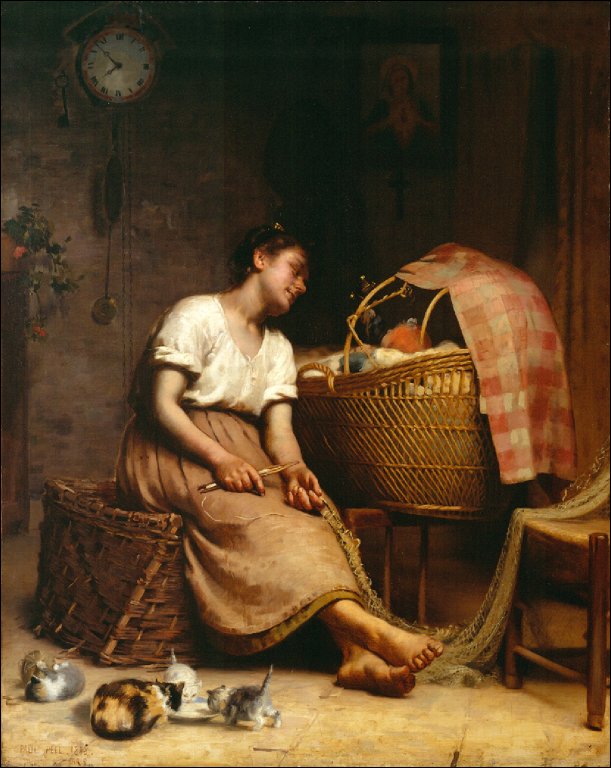This detailed, vintage-style oil painting portrays a humble mother seated in the middle of the composition, seemingly absorbed in the quiet admiration of her baby. Situated beside a wicker bassinet covered with a delicate blanket, the baby gazes up at the mother, creating a tender scene of maternal care. The painting’s color palette includes shades of brown, white, red, gray, and black, enhancing its old-fashioned charm. To the lower left, several playful kittens gather; one engages with a ball of yarn, while three others sip milk from a small saucer. An old clock adorning the background suggests a sense of time gone by, complemented by an image of a saint positioned at the top of the picture, evoking a timeless, almost spiritual, reverence for the depicted domestic bliss. The entire scene is imbued with a cozy warmth that speaks volumes about motherhood and the everyday joys within a modest household.